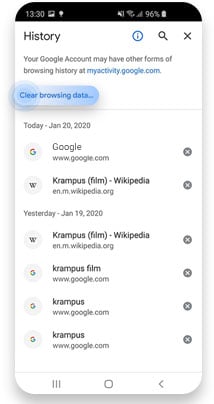### Caption:

A screenshot of a smartphone displaying a webpage is captured in this image. The top section of the screen features a black and white status bar indicating the time as 13:30 (1:30 PM), with a 96% battery charge symbolized by a fully white battery icon. Below this, the page is divided into a couple of sections.

The upper section has a black background with the heading "History" on the left. Underneath, there is a note in black text, informing the user that their Google account may have other forms of browsing history. A blue link labeled "myactivity.google.com" is prominent, followed by another blue link titled "Clear browsing history."

Beneath a thin gray divider line, the day's browsing history is listed, marked with "Today - January 20, 2020":

- **Google**: www.google.com, accompanied by a grey circle with a white 'X' on the right-hand side.
- **Krampus Film Wikipedia Entry**: en.m.wikipedia.org, again with the same grey circle and 'X'.

The history for the previous day, "Yesterday - January 19, 2020," follows:

- **Krampus Film Wikipedia Entry**: en.m.wikipedia.org, with the consistent grey circle and 'X'.
- **Krampus Film Google Search**: www.google.com, similar grey circle with 'X'.

Finally, two more identical entries are listed:

- **Krampus Search**: www.google.com, each accompanied by the grey circle with the white 'X'.

The layout and repeated references to the "Krampus" film indicate a focused browsing activity related to this specific topic over the last two days.